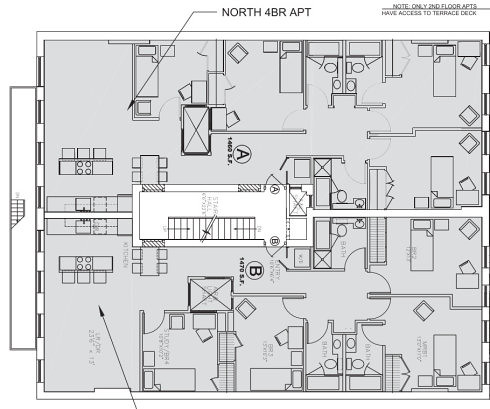Here is a cleaned and detailed caption for the image described:

---

**Architectural Floor Plan of Two Symmetrical Apartments**

The architectural floor plan showcases the layout of two side-by-side apartments, each occupying half of the structure, with a clear division from top to bottom. The entire space is labeled as 'North Floor Bedroom Apartment' and detailed dimensions are provided: the upper apartment (A) measures 1400 square feet, while the lower apartment (B) is slightly larger at 1470 square feet. 

**Apartment A (Upper Unit):**
- **Kitchen and Dining Area:** Located on the left side, the upper apartment features a kitchenette along the bottom wall. There's an island equipped with a four-burner range and three stools. Adjacent to the kitchen is a small dining area with a table and four chairs.
- **Living Space:** Above the dining area is an open space designated for a living room.
- **Bedroom and Office:** To the right of the living space, there is a small bedroom furnished with a single bed, a closet, a desk with a chair, and an additional chair. This room lacks ventilation-related installations, suggesting it may house essential building infrastructure.
- **Bathroom:** A hallway leads to a bathroom that includes a shower, sink, toilet, and bathtub.
- **Additional Rooms:** To the far right of the plan, there is another bedroom equipped with a double bed, a desk, a chair, and a closet.

**Apartment B (Lower Unit):**
- **Entry and Stairwell:** A shared central stairwell provides access, with designated doorways (A and B) leading directly into each apartment.
- **Kitchen and Dining Area:** Similar to the upper apartment, the lower unit also features a kitchenette along the bottom wall. 
- **Living Space and Additional Facilities:** The layout includes comparable arrangements for the dining and living areas, bedrooms, bathrooms, and office spaces, with slight variations in dimensions and furniture placement due to the slightly larger floor space.

A notable feature is the access to a terrace deck, exclusively available to second-floor apartments, as highlighted by a note in the top right corner of the plan. The symmetrical design ensures both apartments share identical structural elements while offering individual, well-appointed living spaces.

---

This caption provides a clear and detailed description of the floor plan, covering key aspects such as room layout, furniture placement, and unique features.